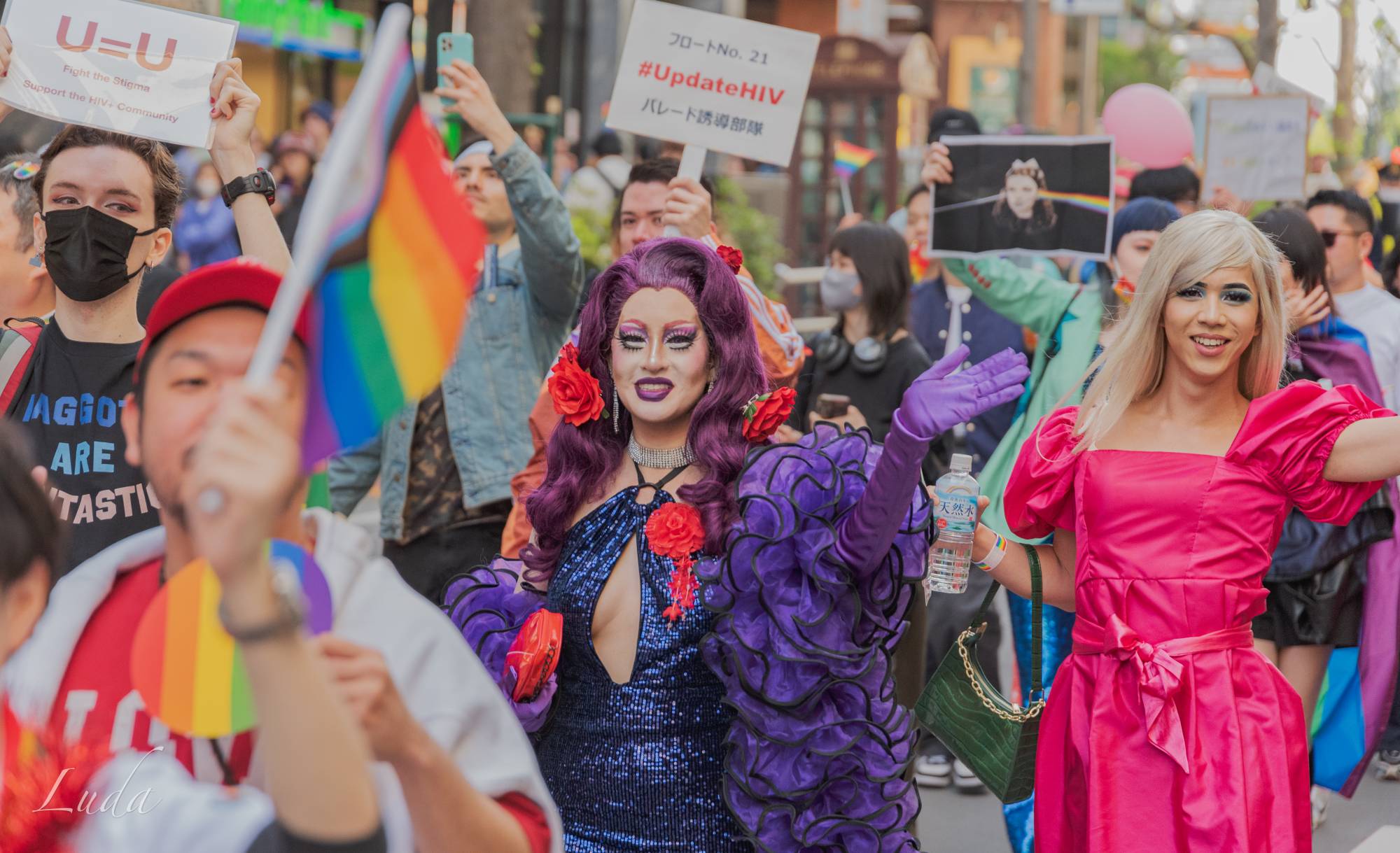In the bustling city, a vibrant gay pride parade unfolds, with participants dressed in an array of rainbow-colored clothing and accessories. The colorful scene is dominated by two central figures: one wearing a glittering, sequined blue evening dress adorned with grand purple ruffles and long purple leather gloves. This person sports long, curly purple hair and dramatic, multicolored makeup. Beside them, a person in a striking bright pink ball gown and puffy sleeves stands out, clutching a green pocketbook and a water bottle. This individual has heavy blue eyeliner and is accompanied by a heavily made-up figure draped in an elaborate outfit and a boa. Around them, a jubilant crowd carries rainbow flags and balloons, with some marching under signs that read “#UpdateHIV” and "U=U". In the background, one participant struggles to capture the moment with their phone as the parade passes storefronts, emphasizing the joyous and inclusive spirit of the event.